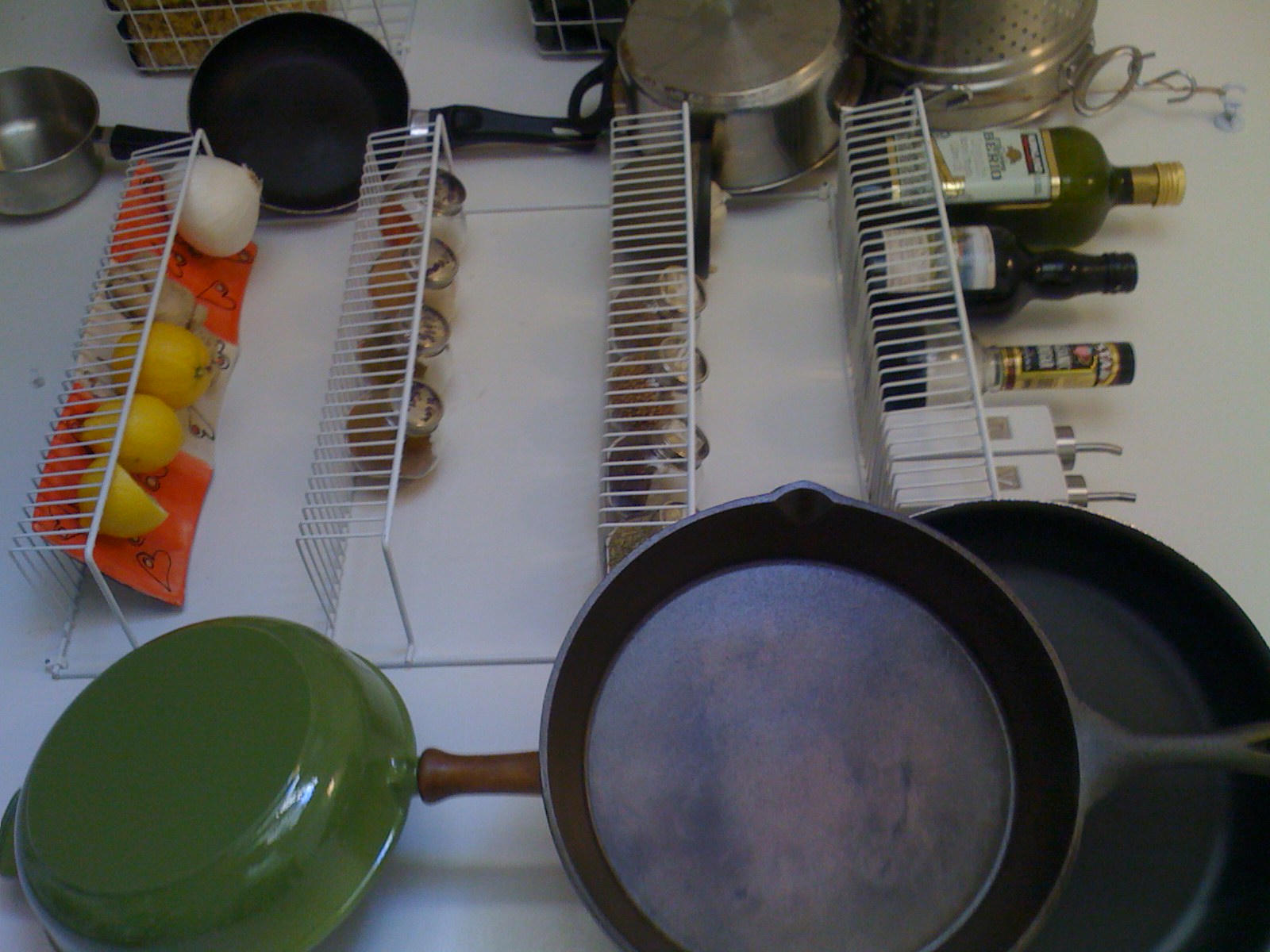This photograph, taken in a kitchen or pantry, captures a neatly organized wire shelving unit turned sideways, with the top of the wall on the right side and the bottom on the left, although the actual top and bottom of the wall are not visible. The shelving unit features four wire basket-like shelves coated in white. 

The bottom shelf is lined with a white and orange tray adorned with heart patterns, holding one onion, a piece of fresh ginger, and two and a half lemons. The shelf above contains four round canning jars with silver lids, each labeled with black sharpie on top. The third shelf from the bottom mirrors the second with additional canning jars and includes a bowl containing a white substance.

On the top shelf, a bottle of Kirkland brand olive oil stands alongside two smaller bottles that appear to contain either oil or vinegar, and two white bottles equipped with silver dispenser tips. 

Framing the bottom of the image are two cast iron skillets and the green exterior of another frying pan. The top edge of the image features various cookware, including a saucepan, a small skillet, a small pot, and a pasta drainer. The background reveals a simple white wall, contributing to the clean and organized aesthetic of the kitchen or pantry space.